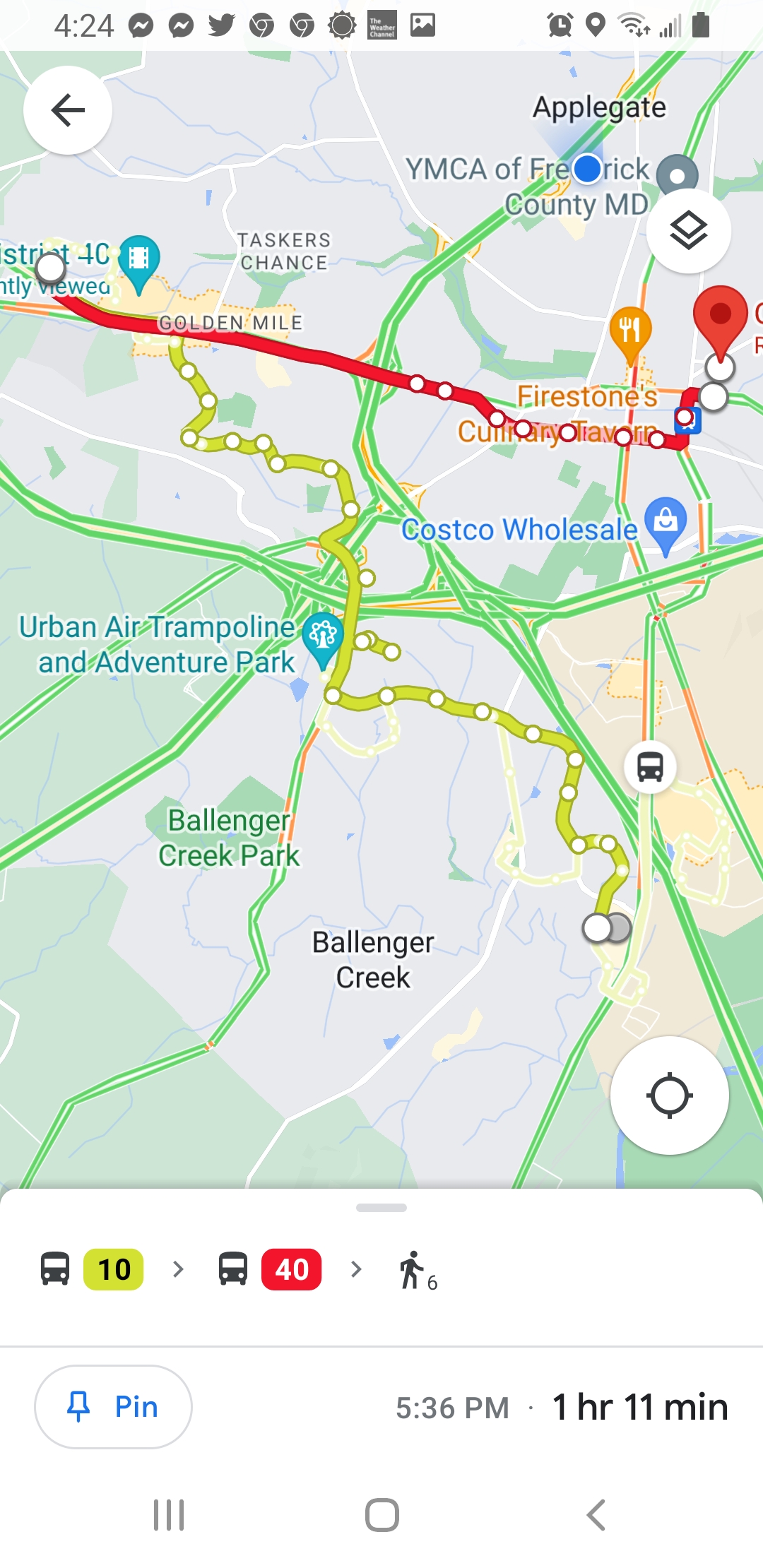This is a colored, portrait-format screenshot of a smartphone displaying a detailed map view from a navigation app, likely Google Maps. The map shows a route from point A to point B, highlighted by a red line connecting the origin and destination. Numerous landmarks and points of interest are marked, including Ballinger Creek, Ballinger Creek Park, Urban Air Trampoline and Adventure Park, District 40, Golden Mile, Tasker's Chance, YMCA of Frederick County, Maryland, Applegate, Firestones, and Costco Wholesale. A bus route is also marked with the first leg in yellow, representing the number 10 bus, followed by a red segment for the number 40 bus, and concludes with a walking route to the final destination. The map visually indicates different traffic conditions with roads in red for heavy traffic, yellow for moderate traffic, and green for light traffic. 

At the bottom of the screen, travel times by bus, transit, and foot are displayed, with a total travel time of 1 hour and 11 minutes. The time stamp is visible, showing 5:36 PM, and typical smartphone status icons like the clock (reading 4:24), Wi-Fi signal, battery strength, and notifications (including a Facebook Messenger message) are displayed at the top.